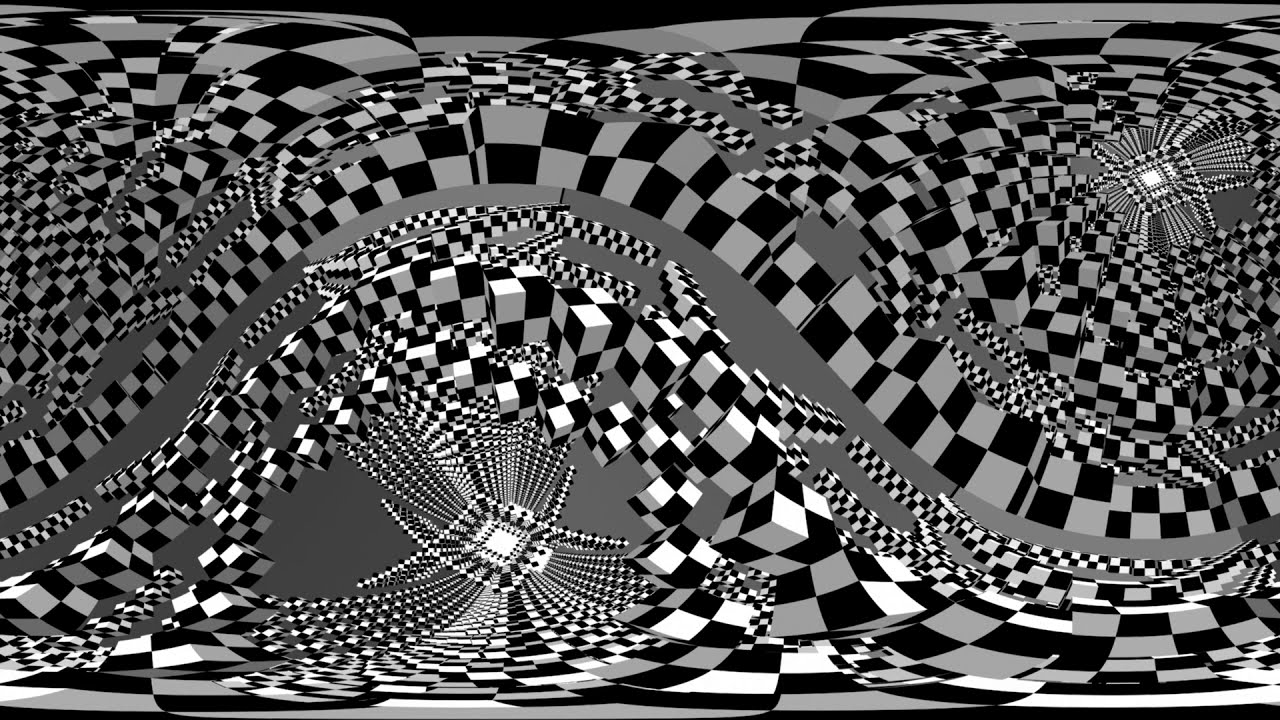This horizontally aligned rectangular image is an abstract, psychedelic graphic design resembling a screen grab from a video. The image features thousands of computer-generated black and white checkered cubes arranged in a fractal-like, vortex pattern. These cubes give the impression of swimming in and out of each other, forming swirling rows reminiscent of a DNA diagram. The pattern, predominantly in gray tones alongside black and white, varies in density and size, starting with densely packed small checks in the upper left corner. Toward the center, the pattern widens into larger checks arranged in gracefully curving rows of gray and black checks stretching from the lower left, across the middle, down to the lower right. This intricate geometric design also includes fine checker patterns towards the bottom left and upper right corners, adding to the chaotic yet mesmerizing composition. Subtle shading and two small white squares in the top right and bottom left add depth, creating an M.C. Escher-like illusion without a definitive light source.